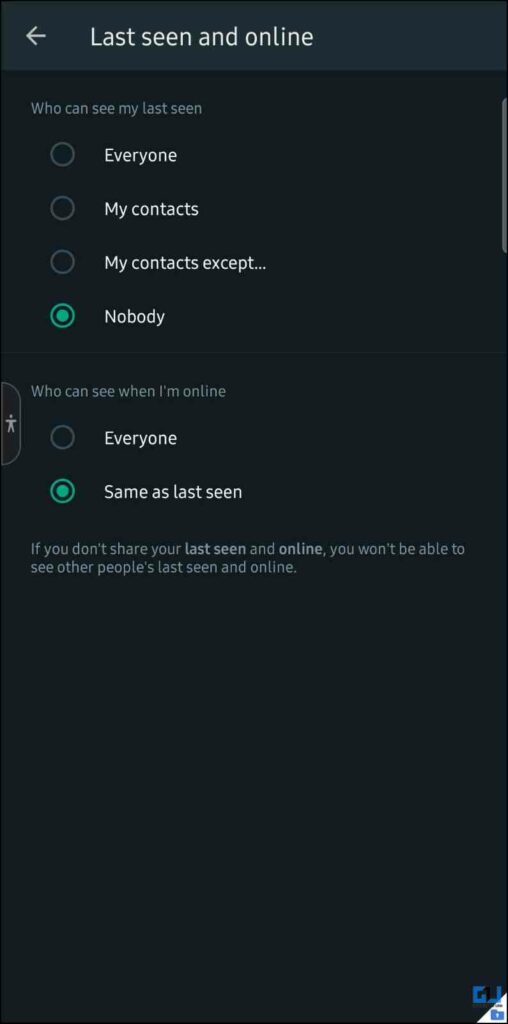This is a detailed screenshot of a smartphone settings page with a focus on privacy options related to online status. The background is black with a slightly lighter black or deep, dark green border. At the top, there's a left-facing arrow and the text "Last seen online." 

Below that, there are option bubbles for "Who can see my last seen" with the following choices in descending order:
1. Everyone
2. My contacts
3. My contacts except…
4. Nobody (highlighted in green)

Underneath these options is a light line separating the next setting. To the left of this line is a person icon next to the text "Who can see when I'm online.” This section has two options:
1. Everyone
2. Same as last seen (highlighted in green)

Below these settings, a note reads, "If you don't share your last seen and online, you won't be able to see other people's last seen and online." On the right side of the screen, there is a scrollbar indicating that there are more settings available if you scroll further down the page.

Overall, this screenshot represents the privacy settings on a smartphone that determine who can view the user's last seen and online status.